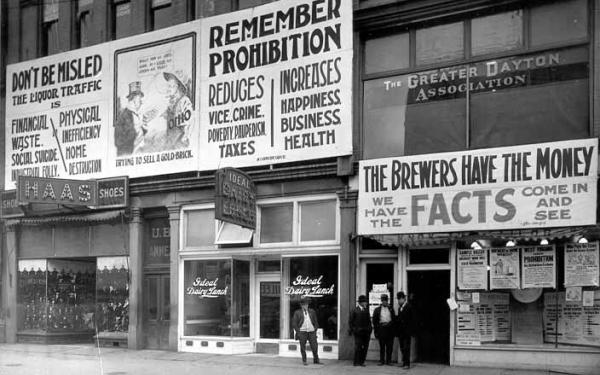This black and white vintage image, possibly from the 1940s or 50s, captures the bustling corner of a city block adorned with tall buildings and numerous advertisements. Dominating the upper portion of the image, a large sign advocates for prohibition, declaring, "Don't be misled. The liquor traffic is financial waste, social suicide, physical inefficiency, home destruction." Adjacent to this primary message is a smaller section featuring an illustration of a man trying to sell a gold brick, accompanied by text that's mostly illegible due to its size. Directly to the right, the sign continues with, "Remember, prohibition reduces vice, crime, poverty, taxes, increases happiness, business, health." Below and to the right, another rectangular sign proclaims, "The brewers have the money, we have the facts, come in and see."

The scene on the street features three storefronts: one with a sign for "H-A-A-S Shoes" on the bottom left, another partially obscured but identified as "Ideal [something]," and finally, "The Greater Dayton Association" with various papers hanging beneath its sign. Four men stand centrally in front of these stores, three clothed in black suits and hats, while one, positioned slightly to the left, wears a gray suit.